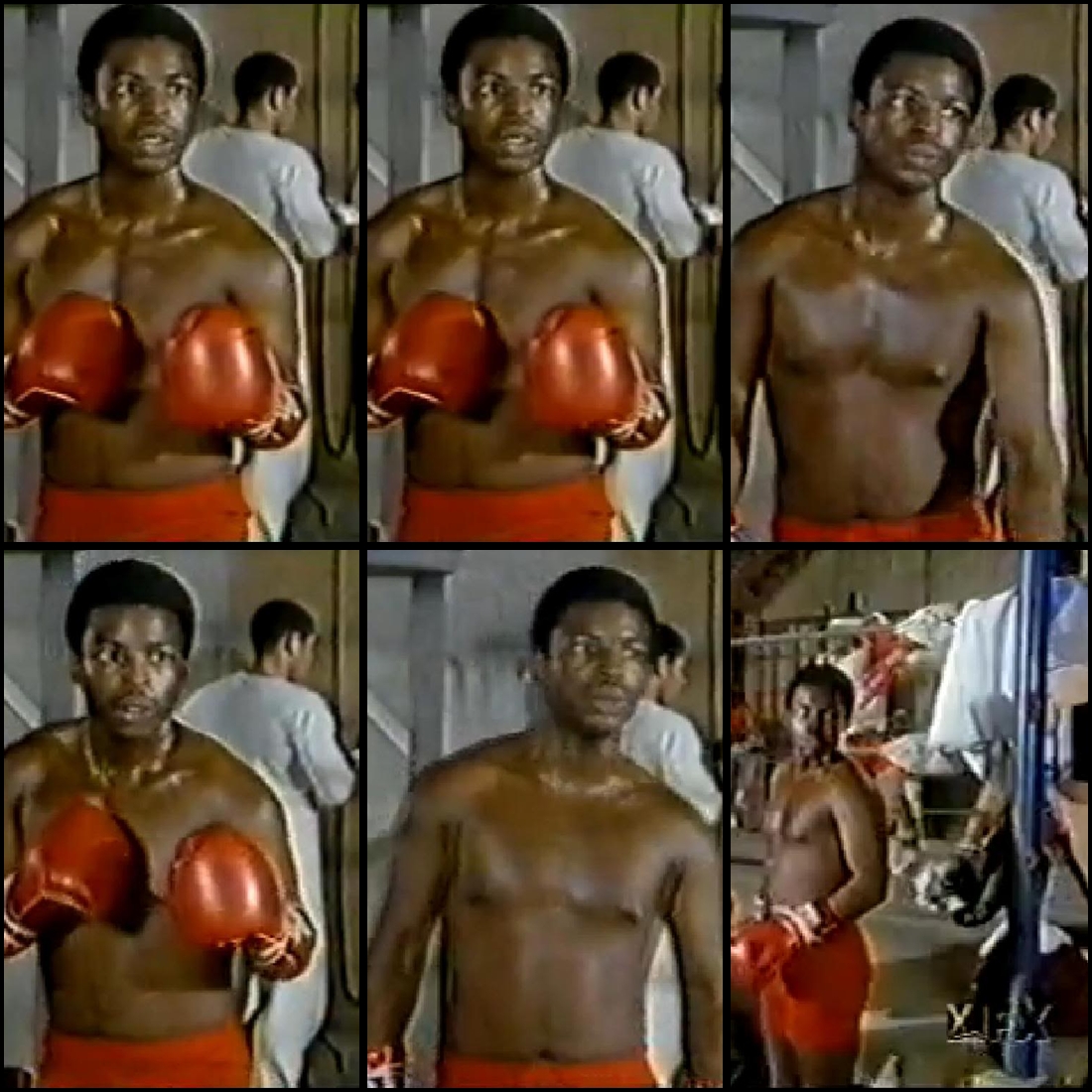The image is a collage of six photographs featuring a young male boxer with short black hair, wearing red boxing gloves and red shorts, while shirtless. The photos are arranged in a 3x2 grid. In the top-left photo, he stands with his red-gloved hands raised in front of him. The top-middle photo shows a similar stance, but with a slight variation in hand positioning. The top-right photo captures him with his hands lowered and head tilted slightly to the side. The bottom-left photo shows him looking aggressive with his hands again raised higher above his chest. In the bottom-middle photo, he stands straight with his hands down by his sides, mirroring the top-right. The bottom-right photo is different; the boxer is angled to the left, looking back towards the camera, with his hands next to his body. A person wearing a white robe is seen in the background of five of the images, and there are clothes or towels visible on the right side of the bottom-right photo.